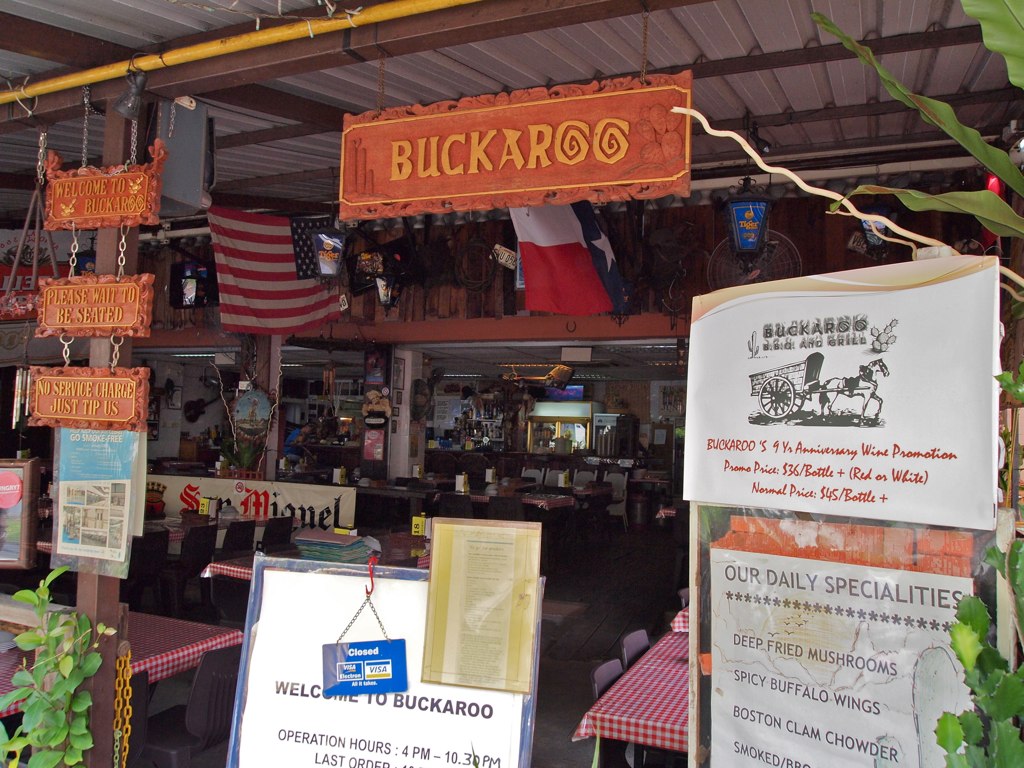This photograph captures the exterior of an outdoor restaurant called "Buckaroo" which features a metal roof. Prominently displayed from the metal rafters is a red wooden sign reading "Buckaroo." Below it, a sandwich board placed on the ground welcomes patrons with the words "Welcome to Buckaroo" and lists the operation hours from 4 PM to 10:30 PM. A red hook on top of the sandwich board holds a closed sign. The interior of the restaurant is adorned with several signs, and all tables are covered with red and white checkered tablecloths. Hanging from the ceiling are two flags, one American and another from a different country. The shop offers a cozy atmosphere, further detailed by a list of daily specials visible inside.